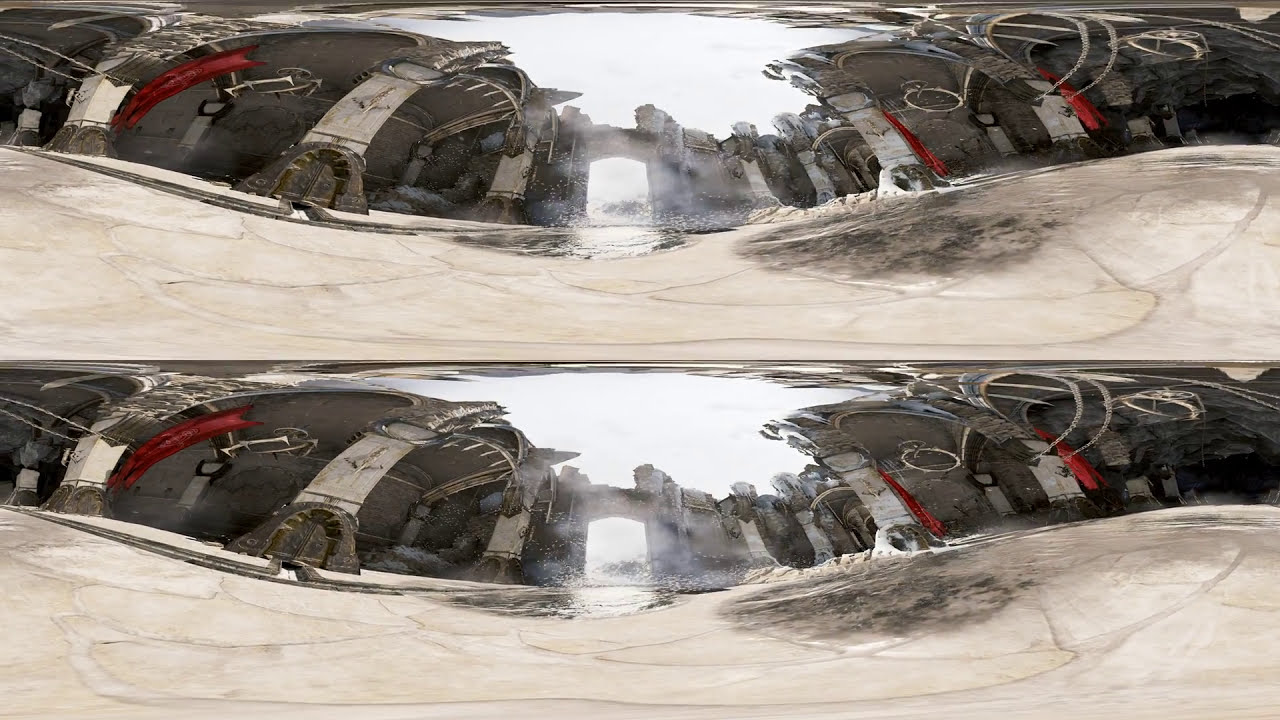The image captures an outdoor setting photographed with a wide-angle lens, creating a curved and distorted effect. It presents two identical photos arranged one above the other in a landscape layout. The scene depicts a seemingly castle-like environment with a prominent stone or concrete archway at the back, which appears lit and serves as a central focal point. The road, which is brown, leads towards this archway. Flanking the road are what appear to be decorative elements resembling red and gray gasoline pumps, two on each side, each adorned with silver squiggles. On the left side, one of these elements is distinctively red and gray. The sky in the background is overcast, emphasizing the gray tones. Adding to the medieval ambiance, there are stone walls lining the sides, adorned with red banners and white-painted beams. Despite the potential real-world setting, the exaggerated distortion of the image suggests a video game-like quality. There is no text within the image.